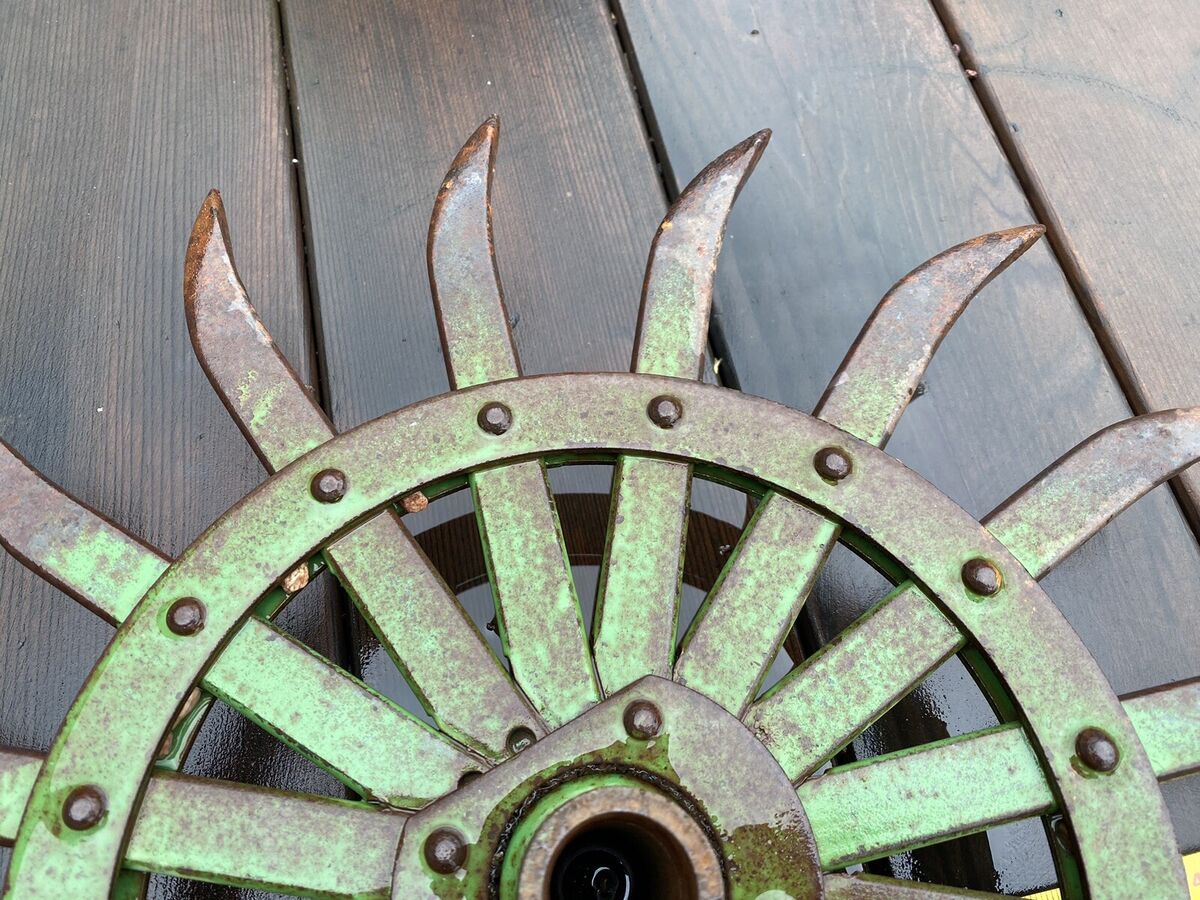This photograph, taken from above, features a half-visible, metal ornamental gear resting on what appears to be wet, brown wooden planks, either flooring or possibly a picnic table. The gear, seemingly handmade and slightly imperfect yet symmetrical, is composed of a patina-shifting, brass-colored metal that is transitioning from coppery tones to a green hue due to oxidation. The central part of the gear includes a circular socket-like hole, and radiating outward are spokes resembling sun rays, each slightly slanted to the right and uniformly rust-stained at their ends. Around the perimeter of the gear, spaced equidistantly, are substantial metal studs or bolts securing an outer concentric circle to the spikes. The gear's weathered, moist surface reflects light, emphasizing its aged, rustic character against the wooden backdrop.